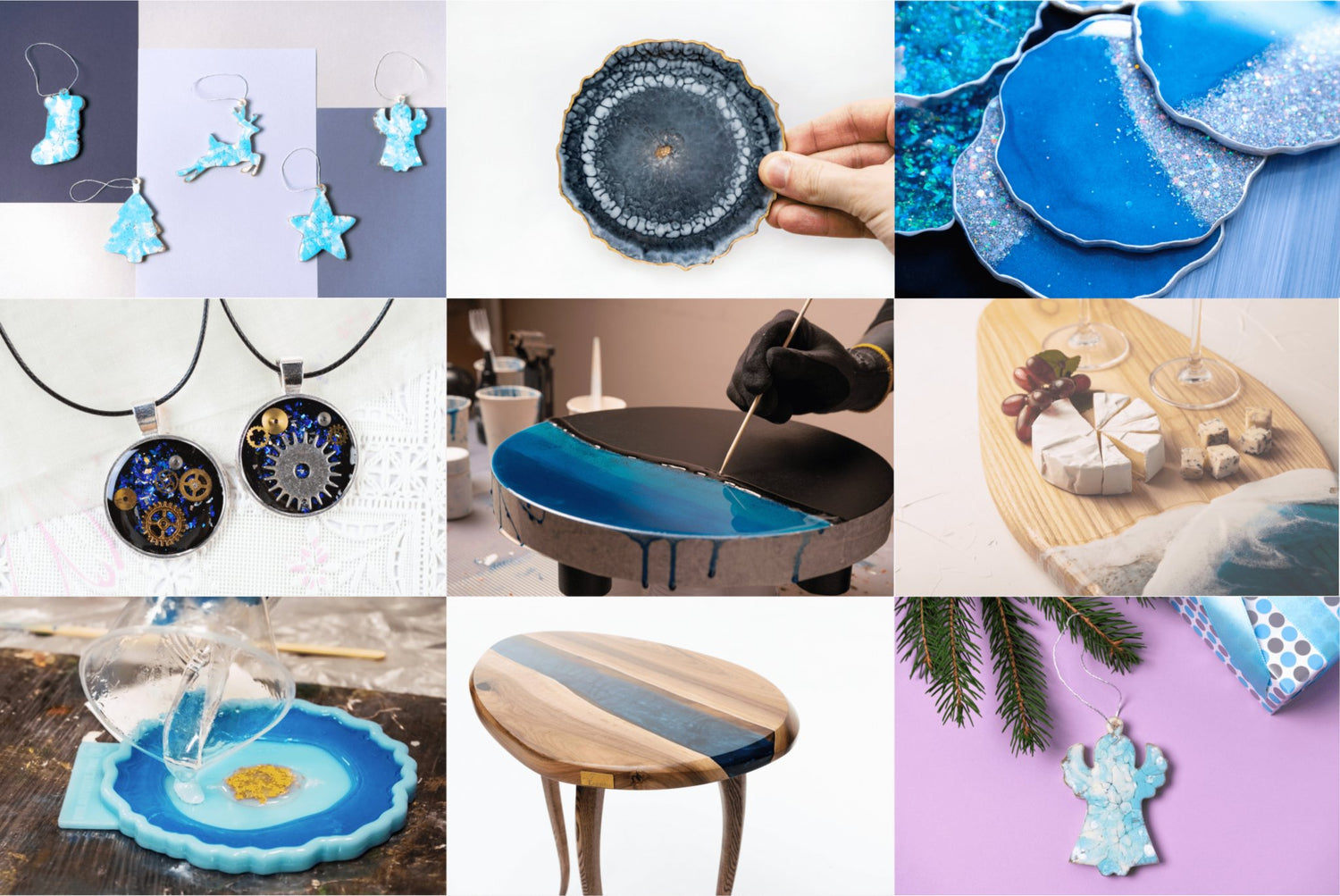The image is a full-color photograph comprised of a collage of nine distinct, staged photographs, all with a common blue theme and no overall border but clear separations between them.

1. **Top Left**: Features several blue, shiny Christmas ornaments, including shapes like a stocking, tree, reindeer, star, and angel, arranged over a background of blue squares.
2. **Center Left**: Displays two circular, gear-like objects on necklace chains with intricate designs, primarily in gold and blue.
3. **Bottom Left**: Shows a blue dish covered by a clear lid.
4. **Top Center**: Contains a small, blue-and-white dish that resembles a coffee saucer.
5. **Center**: Captures a person in black gloves painting the top of a table that is half blue and half black.
6. **Bottom Center**: Depicts a wooden table with a varnished, dark strip running along the middle.
7. **Top Right**: Shows a set of blue, shiny and sparkly Christmas ornaments.
8. **Center Right**: Presents a charcuterie board with grapes and assorted cheeses, along with the contrasting element of a chartreuse-colored board underneath.
9. **Bottom Right**: Includes a small blue Christmas ornament shaped like an angel, accompanied by pine branches and set against polka dot paper on a purple background.

The collage as a whole highlights the meticulous arrangement and the prevalent use of blue hues in various objects, enhancing a festive and detailed visual narrative.